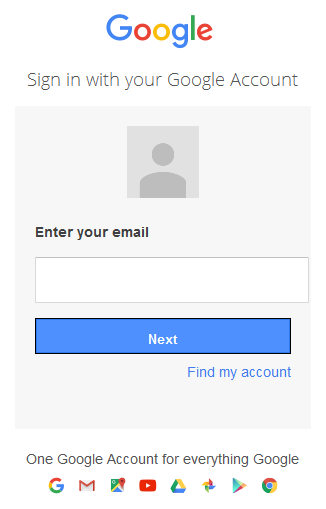The image depicts a Google sign-in page. At the top, there's a simple Google logo, composed of the word "Google" in multi-colored letters: blue, red, yellow, blue, green, and red. Below the logo, dark gray text prompts the user to "Sign in with your Google account."

Centered on the page, there's a sign-in box featuring a default user icon, which is a generic human figure silhouette, signifying that no custom user icon is available or the user has not yet signed in. Directly beneath the icon, a black text label reads "Enter your email," accompanied by an empty text field for the user to input their email address.

Further down, a prominent blue button with white text marked "Next" is provided to proceed with the sign-in process. Just below this button, a blue link reads "Find my account" for users needing assistance.

At the bottom of the page, a message in black text states, "One Google account for everything Google," followed by icons representing various Google services such as Gmail, Maps, YouTube, Google Drive, and Google Chrome.